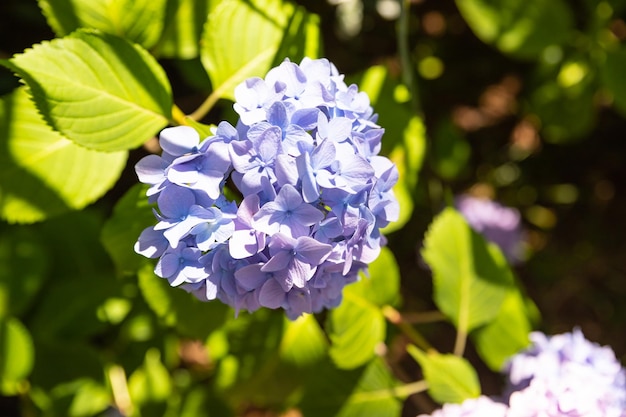A vibrant, outdoor photograph captures a striking close-up of a violet-blue hydrangea bloom, hanging prominently in the center of the frame. This main flower boasts four-petaled blossoms forming a compact, dome-shaped cluster, set against a backdrop of verdant, serrated green leaves. The vivid green leaves are a lush, rounded contrast to the intricate flowers, filling much of the image and creating a dense, natural tapestry. Although the background remains blurred, hints of lavender and bluish-purple hydrangeas peek through, with additional clusters subtly visible along the bottom-right edge. The sunlit scene bathes the details in warmth, highlighting the contrast between the sharp focus of the primary bloom and the soft, indistinct shapes behind it.